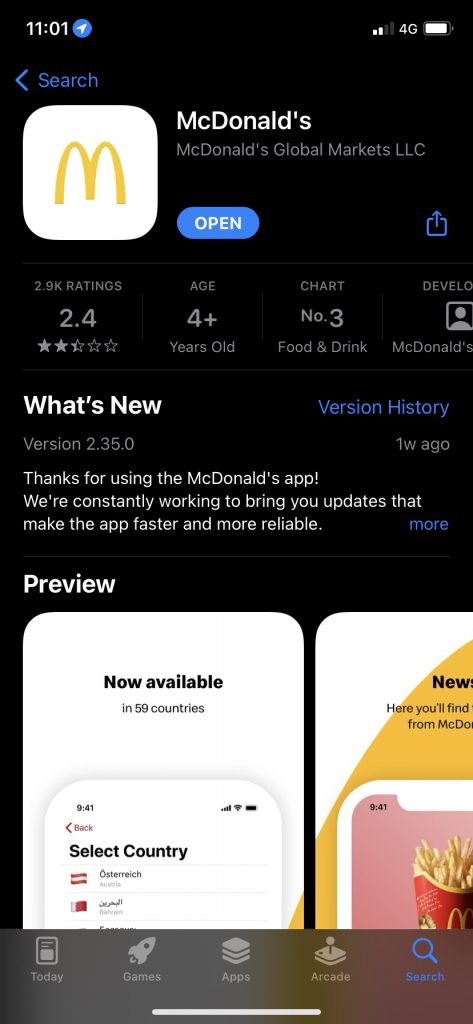A detailed screenshot depicting a mobile phone interface is observed in this image. At the very top, there is a horizontal black bar, featuring the time "11:01" in the upper left corner. Adjacent to the time, within a blue circle, there is a white arrow point in a direction, likely indicating navigation. In the upper right corner, connection status icons are visible, including indicators for 4G internet and the current battery level.

Directly beneath this black bar, a white search bar is present with the text "Search," accompanied by a leftward-facing arrow under the time.

Central to the screenshot is a white box displaying the McDonald's logo—a yellow "M"—with the adjacent text "McDonald's Global Markets LLC" in white. Below this, there is a blue oval button labeled "Open," suggesting an actionable link to engage with the McDonald's app. Alongside, the app's summary reveals a rating of 2.9 stars, an age rating of 4+, and the current version "2.35.0". A "version history" link is also visible.

The app's details say, "Thanks for using the McDonald's app. We're constantly working to bring you updates that make the app faster and more reliable." Further content includes a preview section with a white rectangle, stating the app is now available in 59 countries. Adjacent visuals include images likely representing the app interface, one featuring a red box of McDonald's fries.

At the bottom of the screenshot, the phone's icon bar is partially visible, showing the sections "Today," "Games" (represented by a spaceship icon), "Apps," "Arcade" (with a game controller icon), and a "Search" option symbolized by a magnifying glass.

Overall, the screenshot provides a thorough view of the McDonald's mobile app listing as seen on a user's phone interface, emphasizing its current version, functionalities, and user interface visuals.